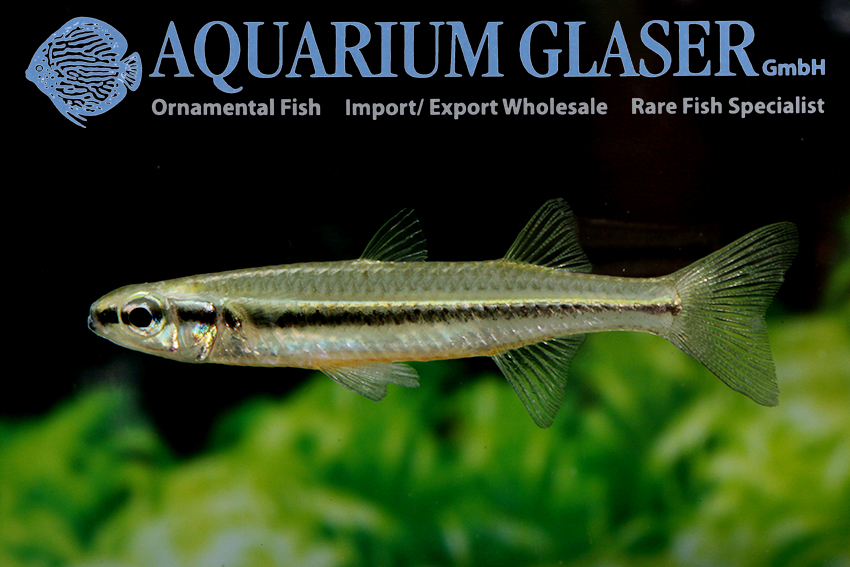The image predominantly features a long, slender, and almost translucent ornamental fish, characterized by its silvery hue and a striking black stripe that runs the length of its body, from mouth to tail, which fades slightly at the end. The fish has a distinct side profile showcasing a dark eye and a combination of fins: two sets in the midsection (one pair on the top and one pair underneath) and a tail fin. It appears to be swimming in water blurred out in the background, which hints at green vegetation below, indicating the presence of aquatic plants. At the top left corner of the image, there is a blue outline of an angelfish beside bold blue text that spells "Aquarium Glaser GmbH." Underneath, in white text, the words "Ornamental Fish, Import/Export, Wholesale, Rare Fish Specialists" detail the services offered by Aquarium Glaser.